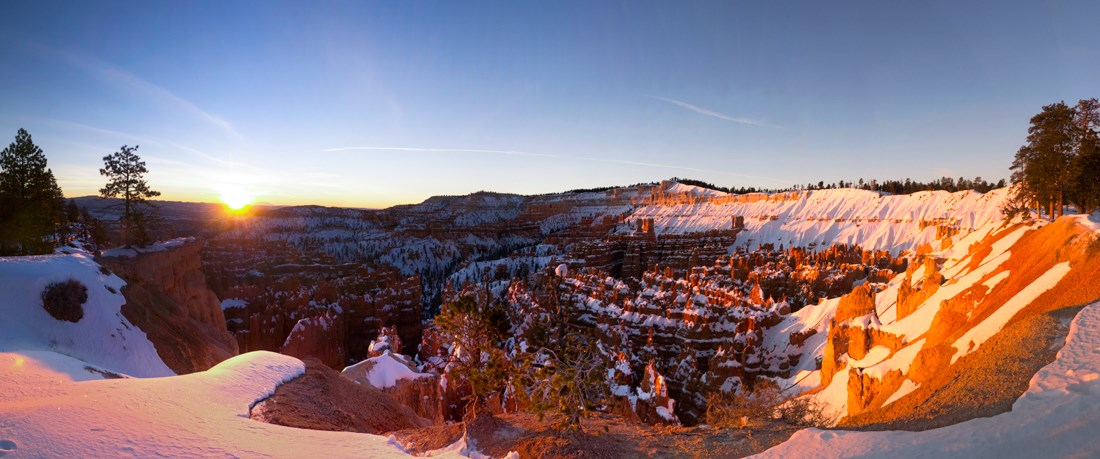The image showcases a breathtaking winter landscape of a snowy canyon during sunset. The snowy gorge is bathed mostly in shadow, with sunlight illuminating areas along the right edges and the center. Green bushes without any snow dominate the immediate foreground. To the left, a few trees, including pines, add depth to the scene, while a large forest can be seen in the background on the right. The rugged canyon floor is dotted with small, partially snow-covered rock spires, creating a dramatic contrast against the predominantly shadowed environment. The top portion features a bright blue sky streaked with clouds, with the sun just peering over the rocks, casting a golden hue and reflecting light onto the snowy peaks. The steep, rocky embankments culminate in jagged points, creating a picturesque and serene winter vista.